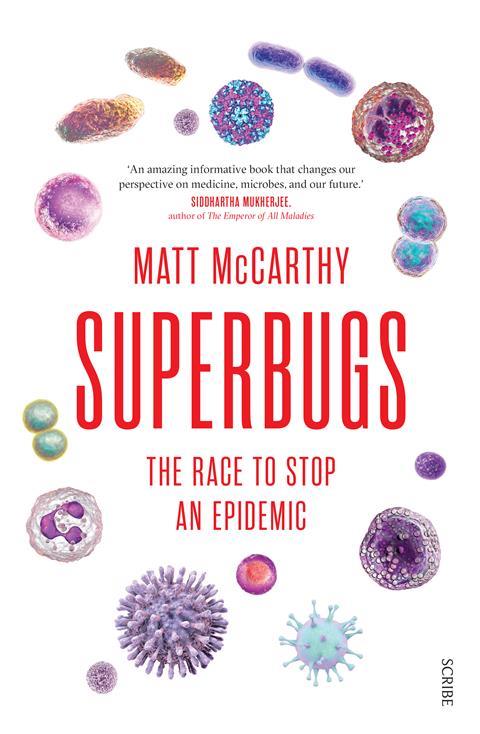The book cover of "Super Bugs: The Race to Stop an Epidemic" by Matt McCarthy features a striking design centered around its bold, bright red title, "Super Bugs," which spans the middle of the cover in capital letters, making it the focal point. Above the title is the author's name, also in red but in a smaller font, "Matt McCarthy." A subtitle, "The Race to Stop an Epidemic," appears just below the main title. At the very top, there is a laudatory blurb: "An amazing, informative book that changes our perspective on medicine, microbes, and our future," by Siddhartha Mukherjee, author of "The Emperor of All Maladies." The entire cover is adorned with various colorful images of stylized microbes and cells in shades of purple, green, blue, and occasional yellow, some spiky and some smooth, giving it a dynamic and vibrant look. In the bottom right corner, the name "Scribe" indicates the publisher. The white background effectively enhances the prominence of both the text and the colorful microbial imagery.